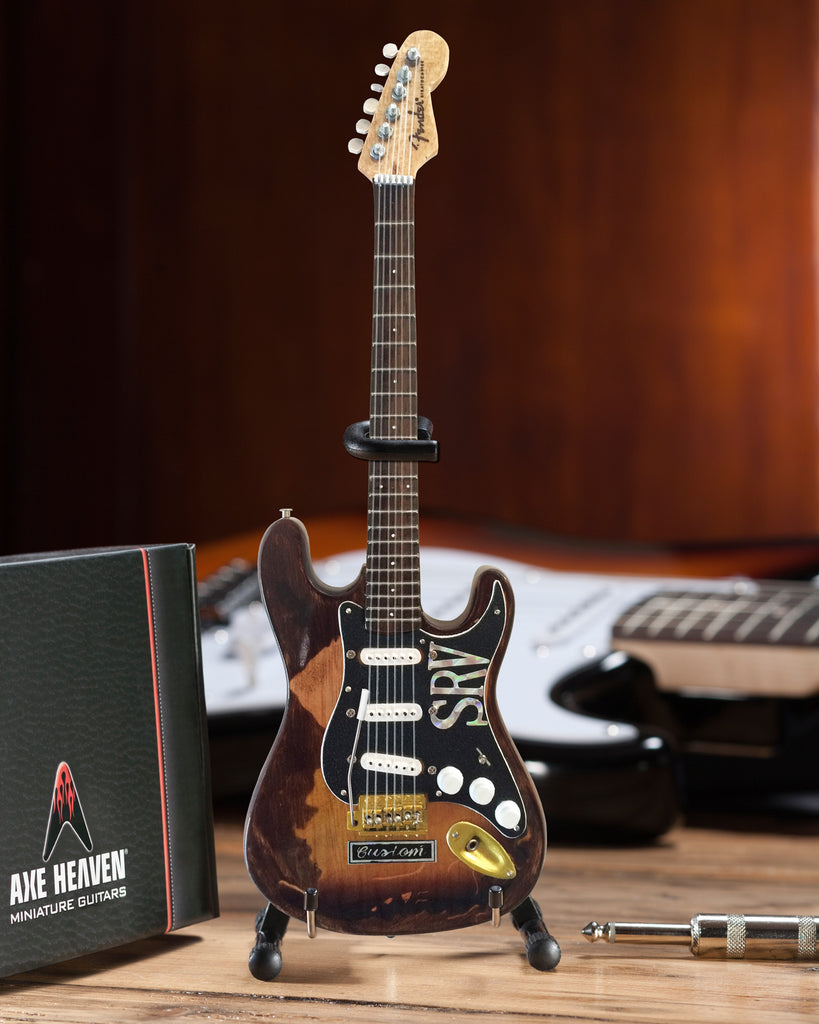This image depicts a miniature guitar prominently displayed on a light-colored wooden desk or counter, with a wooden wall as the backdrop. The miniature guitar, emblazoned with "SRV" in reflective silver text, features a light wooden top contrasted with a darker brown neck and weathered-looking dark brown body. Notable details include a black panel behind the pickups, several white knobs, and a golden area for the plug-in. The guitar rests on a black miniature stand, which has silver extensions with rubber grommets for support. Accompanying the guitar is a box labeled "Axe Heaven Miniature Guitars" on its left side, marked by red stripes. An auxiliary cable for size comparison lies next to the guitar, emphasizing its small scale. In the background stands a regular-sized guitar with distinctive white paneling and a brown tone, adding further context to the size of the miniature replica.